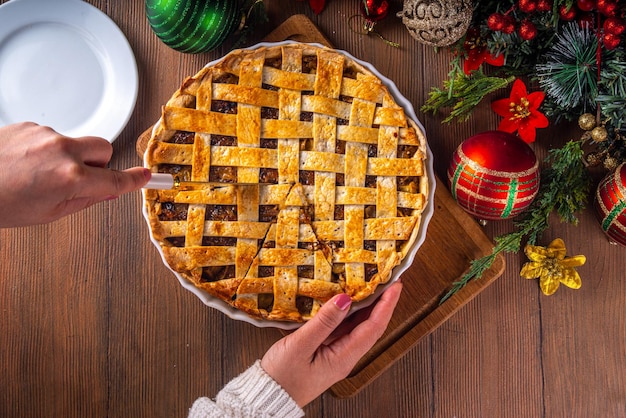The photograph captures a festive scene of a pie being served. Someone is in the process of cutting a second slice of the pie with a knife, while one slice has already been removed. The pie features a distinctive lattice crust that has been carefully woven over the top, suggesting it might be a fruit pie, possibly apple, as pecan pies typically do not have a lattice topping. The interior of the pie has a brownish hue, which could indicate a dark golden filling. Surrounding the pie, the scene is adorned with Christmas decorations, including red, green, and possibly yellow ornaments, evergreen tree branches, and small poinsettia flowers, enhancing the holiday spirit.